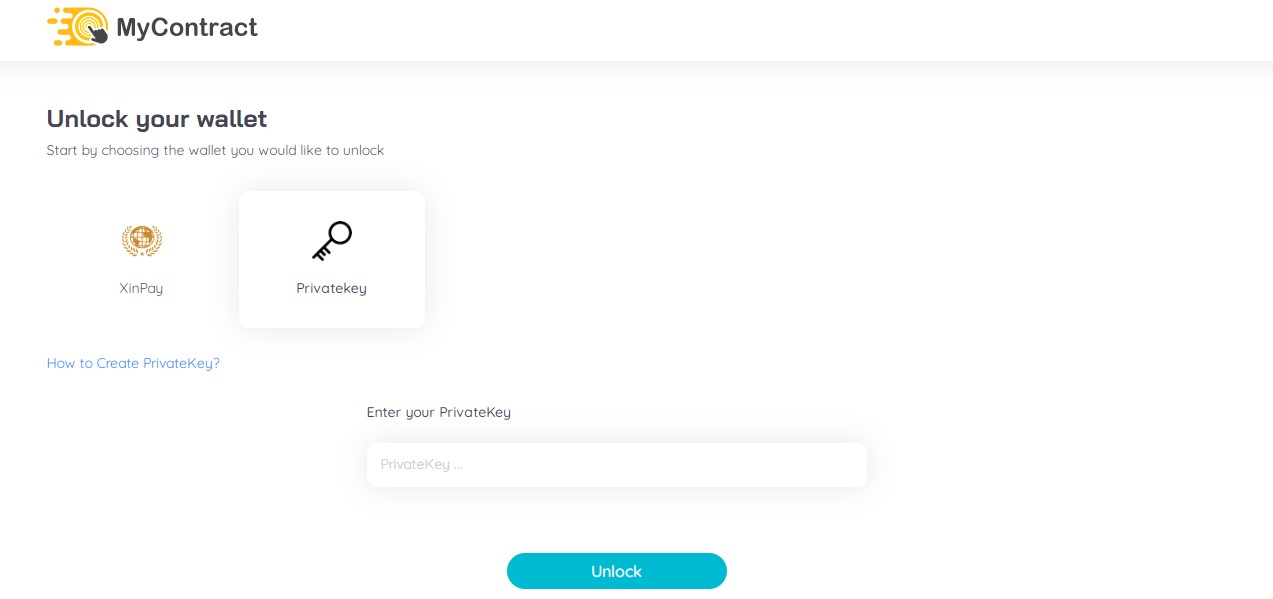The image appears to be a screenshot of a computer interface related to unlocking a digital wallet. In the upper-left corner, it features the text "My Contract" accompanied by a circular symbol. This symbol is a yellow circle emitting watery flame-like shapes from its left side, with a black hand and finger pointing towards its center. Below this, a light gray line spans across the screen. The text "Unlock Your Wallet" is prominently displayed in black, with a smaller gray text stating "Start by choosing the wallet you would like to unlock."

Underneath this instruction, there are two selectable options presented as squares. The first option, labeled "Zin Pay," features a symbol resembling that of the United Nations. The second option, labeled "Private Key," displays a black skeleton key icon. The "Private Key" option appears to be selected, as it is bolder than the other.

In the lower center of the image, there is a large, horizontal white box labeled "Enter your private key" with placeholder text inside that reads "Private key." At the very bottom center of the screen, a teal-colored horizontal oval button is labeled "Unlock," which is likely intended to be clicked on to unlock the wallet after entering the private key.